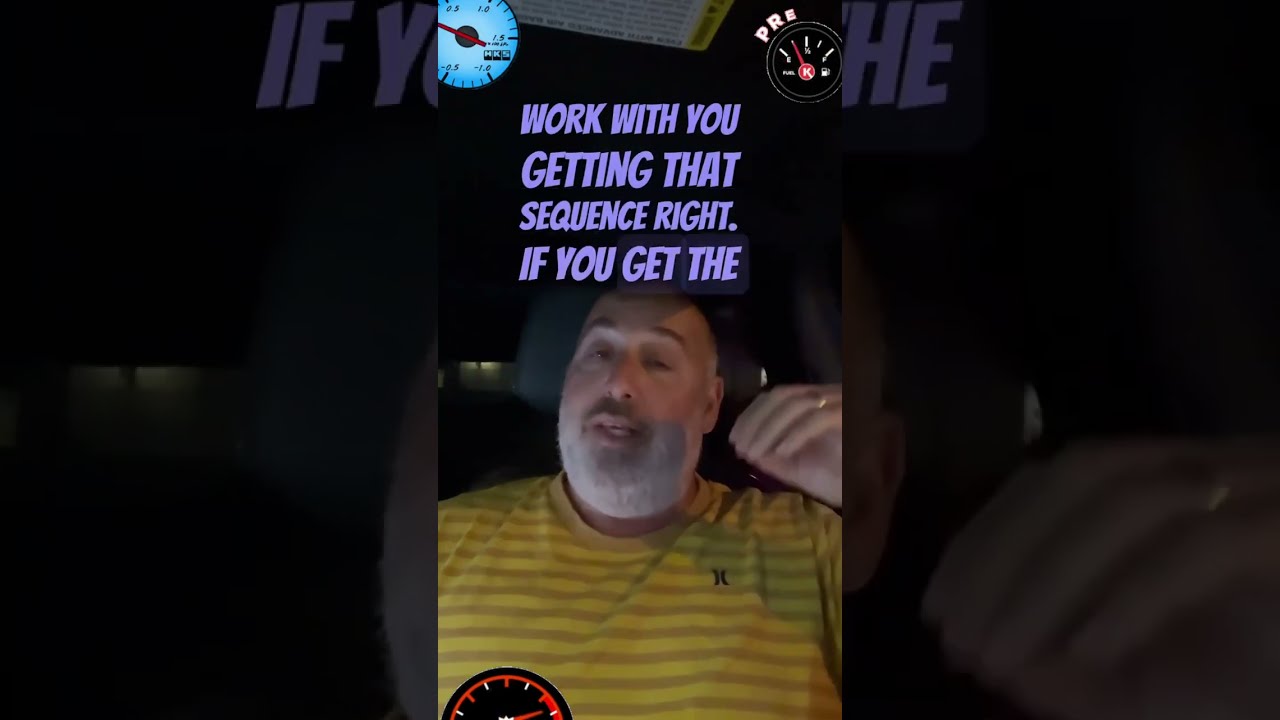The image showcases a layered, composite photograph, likely from a smartphone, where a central focus is a man sitting inside a car at night. The man, who is bald and has a very short gray beard, appears to be speaking with his mouth partially open. He's dressed in a gold and yellow striped t-shirt, identified as possibly by the brand Hurley, and wears a gold wedding ring on his left hand. In the middle above his head, there is text in purple font that says, "work with getting that sequence right if you get the..." which gets cut off, suggesting a transition to another part of a story or reel, typical of Instagram or TikTok. Behind him, a headrest is visible, and the darker background indicates the setting is night. The image also includes superimposed elements such as a speedometer with a light blue background and a red needle in the upper left corner, and a fuel gauge icon labeled "P-R-E" in white letters on the upper right. These instruments seem digitally altered into the picture for artistic effect. The photograph's darkened, faded-out edges create a framed or bordered look, enhancing the central scene.